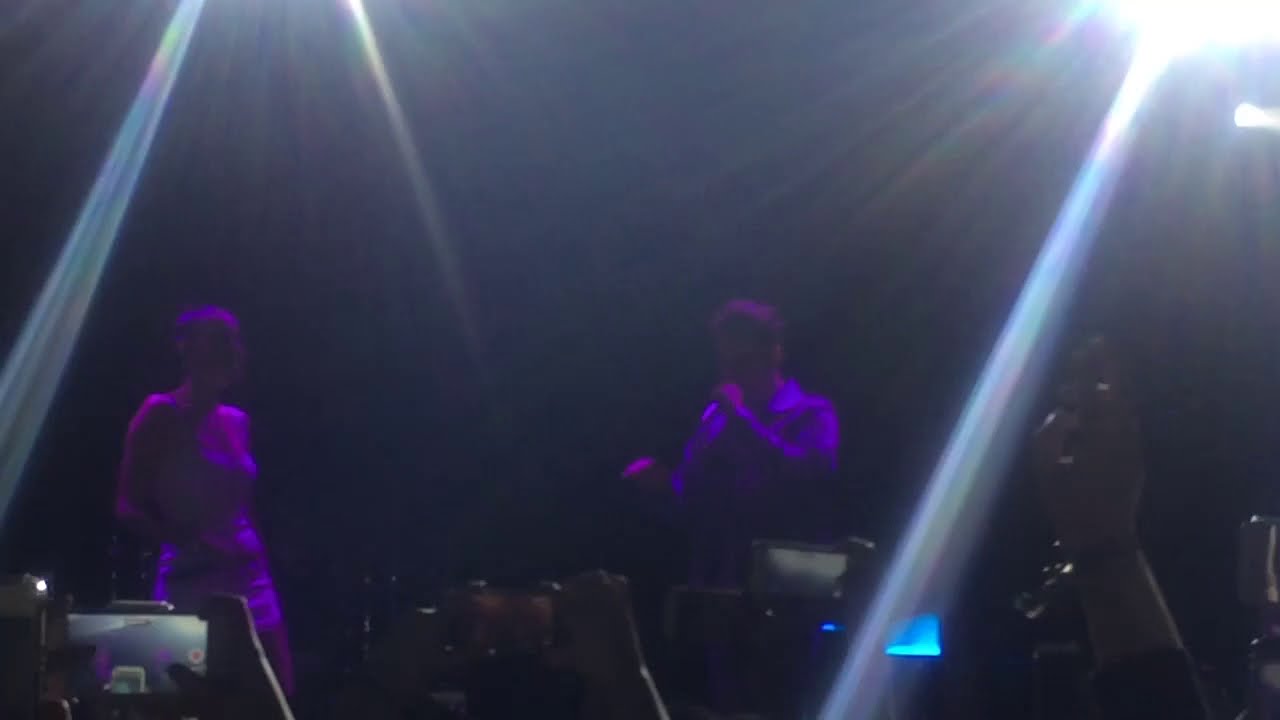The image captures a dimly lit, indoor concert or nightclub scene with a male singer on stage, holding a microphone, and seemingly either talking or singing. He wears a long-sleeve, collared shirt, which appears to be purple. Next to him stands a woman with short hair, dressed in a sleeveless, very short white dress. The stage is illuminated by bright lights, possibly strobe lights, which contrast sharply with the very dark background. The audience, partially visible, holds up phones and cameras, recording or taking pictures of the performance. The photo quality is poor, blurry and dark, obscuring many details and offering no identifying information about the venue, date, or location.